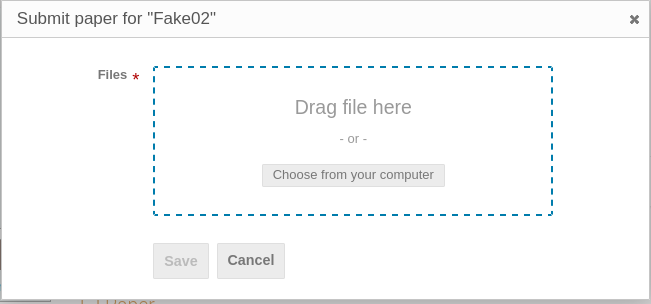**Caption:**

Under the heading "Websites," the interface showcases a streamlined design intended for submitting papers. At the top, a light gray bar spans horizontally, displaying the text "Submit Paper for 'Fake 02'," with an 'X' at the far right corner to close the section. Below, a larger white box is prominently featured, titled "Files," accompanied by a red star indicating a required field. Inside this box, a blue dashed rectangle is presented with the instruction "Drag file here – or –" flanked by hyphens. Below this instruction, a gray rectangle with the label "Choose from your computer" provides an alternative file-uploading method. Further down, options to "Save" or "Cancel" your action are available. A gray bar beneath these options contains indistinct text due to its condensed presentation. Notably, the gray borders along the bottom are thicker compared to those at the top and sides, emphasizing the footer area. Overall, this interface serves as a concise and organized submission form likely intended for uploading document files.